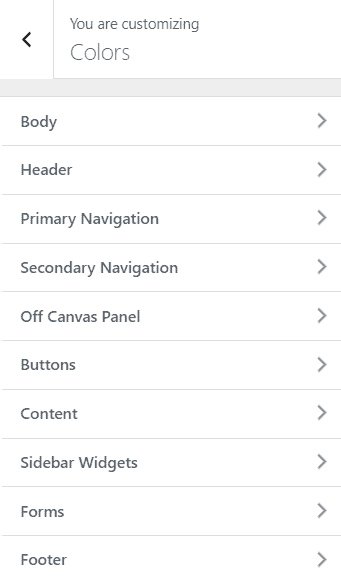In the image, a user is navigating a color customization section within an app's settings. The screen displays options for adjusting colors for various web page elements, including Body, Header, Primary Navigation, Secondary Navigation, Off-Canvas Panel, Buttons, Content, Sidebar Widgets, Forms, and Footer. The background of this settings area is white, with black text for clear readability. There is a notable back button, allowing the user to return to the previous settings page. Each listed element likely opens additional settings for detailed color customization, possibly involving hexadecimal color codes or a more intuitive color selection system. An arrow suggests that clicking on an element, such as Header, will reveal more specific options for changing its color. This section appears focused on providing comprehensive control over the visual appearance and placement of UI elements on the web page.